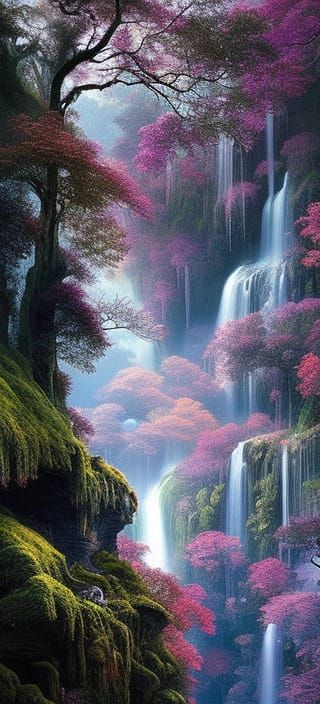This is a detailed, vertically-oriented artwork that appears to be a drawing, painting, or possibly a low-resolution CGI image, replicating a fantastical forest landscape. The composition features very tall trees growing out of a rocky terrain with lush, green moss. The foliage and flowers adorning the trees are vibrant shades of purple, pink, and red. On the left side, trees with green branches extend towards the center, while the right side is dominated by the cliffs from which multiple waterfalls cascade. These waterfalls are numerous, flowing from the top of the cliffs down to various points, creating a mesmerizing web of water streams. The scene is lit by daylight, with glimpses of sky and sunlight peeking through the canopy. The overall effect is a stunning, dreamlike environment that blends lush greenery with vivid floral accents and dynamic water elements.